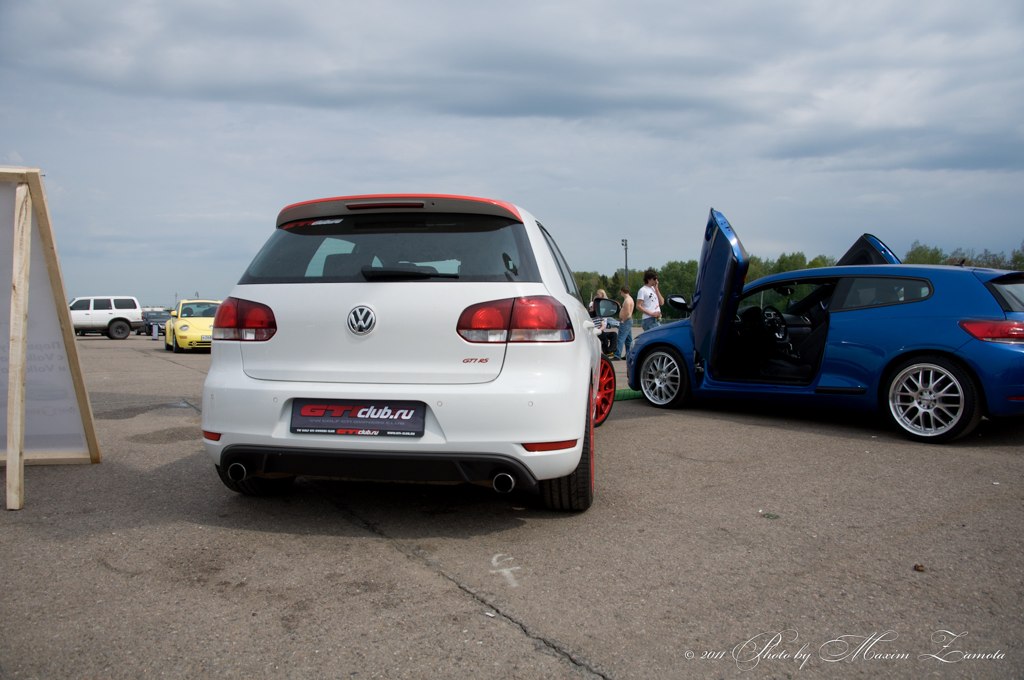The photo depicts a car meet in a large, open parking lot under a completely overcast, gray sky. Dominating the scene is a white Volkswagen GTI hatchback situated towards the left side of the image. This vehicle is identifiable by its VW logo and a unique license plate tag reading "GTI club.ru," with "GTI" in red and "club.ru" in white. The car features red trim and red engine details along with black tires, creating a prominent contrast. 

To the right of the Volkswagen, there is a striking dark blue two-door sedan characterized by its silver chrome rims and distinctive winged doors that open upwards. The two cars are angled towards each other at approximately 45 degrees. In addition to the main cars, the background reveals several other vehicles, including a yellow car and a white SUV. People are milling around, many of them intrigued by the blue sedan, while others are seen further back inspecting another vehicle. 

The parking lot itself is a light gray concrete or asphalt surface with noticeable cracks. On the far left, there is a wooden sign mounted on 2x4s, positioned away from the photographer. In the lower right corner of the photo, there is faint text that reads, "2011 photo by Maxim Lanola," although it appears slightly blurry. The overall atmosphere is one of an enthusiastic car gathering despite the cloudy weather.